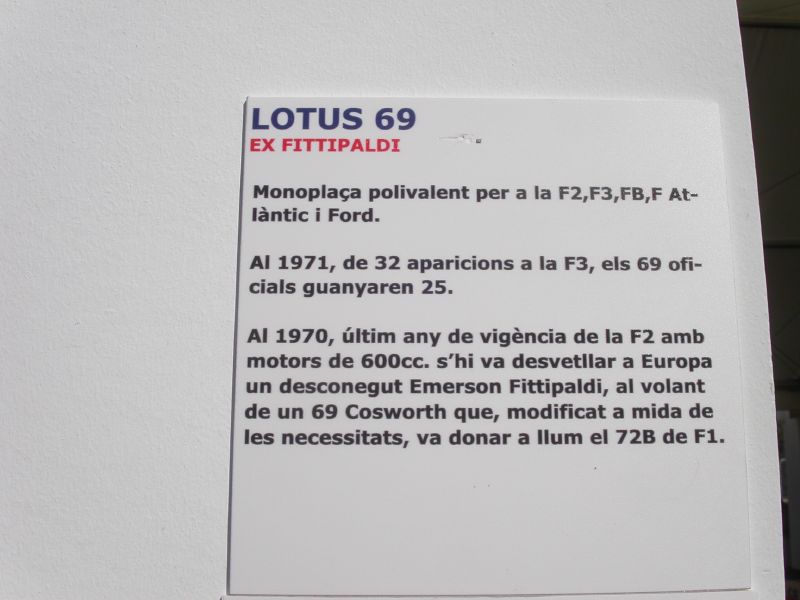The image depicts a color photograph featuring a piece of paper with detailed inscriptions related to the Lotus 69 car, specifically linked to the Ford company and the Atlantic I Ford. The paper itself is a smaller square or rectangular piece, occupying about three-quarters of the height and width of the photograph, and sits atop a larger greyish-white sheet. Both pieces of paper appear to be placed on a background that includes a narrow, ridged, black triangular shape running vertically on the left side. The top of the smaller paper prominently displays the text "Lotus 69" in large, very dark blue ink, followed by "Ex Fittipaldi" in red ink. Below this, three paragraphs of text are written in black ink, possibly in French or Spanish, consisting of brief lines that include technical specifications and historical data. The first two paragraphs contain a line and a half of writing each, while the final paragraph extends to five lines.